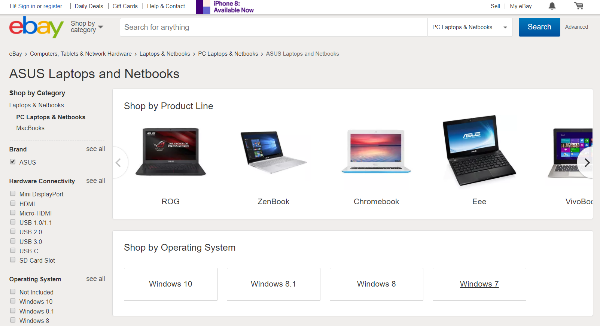This is a detailed screenshot of the eBay website's interface, specifically highlighting a section focused on various laptops and notebooks. 

At the very top of the webpage, there are two graph-like lines, one purple and one blue. To the right, a purple banner announces "iPhone 8 available now." In the top-right corner, there is a cluster of icons and text: the word "Sell," some illegible text, a gray notification bell, and a gray shopping cart.

The top portion of the page has a gray background. On the upper left side, the colorful eBay logo is prominently displayed, followed by the text "Shop by category" in black, accompanied by a downward arrow. Next to this, on the right, there is a blank search input area with some broken, unreadable text to its right. On the far right of this section is a blue rectangular button that says "Search" in white.

Beneath this top section, there is a header reading "Asus laptops and notebooks." A vertical sidebar on the left lists various categories in black text: "Shop by category" and "Brand," with "Asus" being checked off. Other partially visible categories include "Hardware connectivity" and "Operating system."

On the right-hand side, there are two rows of information on a white background. The uppermost row displays a series of laptops arranged horizontally. The top left corner of this white section reads "Shop by product line" in black. Featured laptops include a black laptop labeled "ROG," followed by models named "ZenBook," "Chromebook," something resembling "EBO," and a "VivoBook." Navigation arrows for browsing more images are positioned to the left and right.

At the bottom of the white section, the text "Shop by operating system" appears in the upper left corner in black, followed by four options: Windows 10, Windows 8.1, Windows 8, and Windows 7.